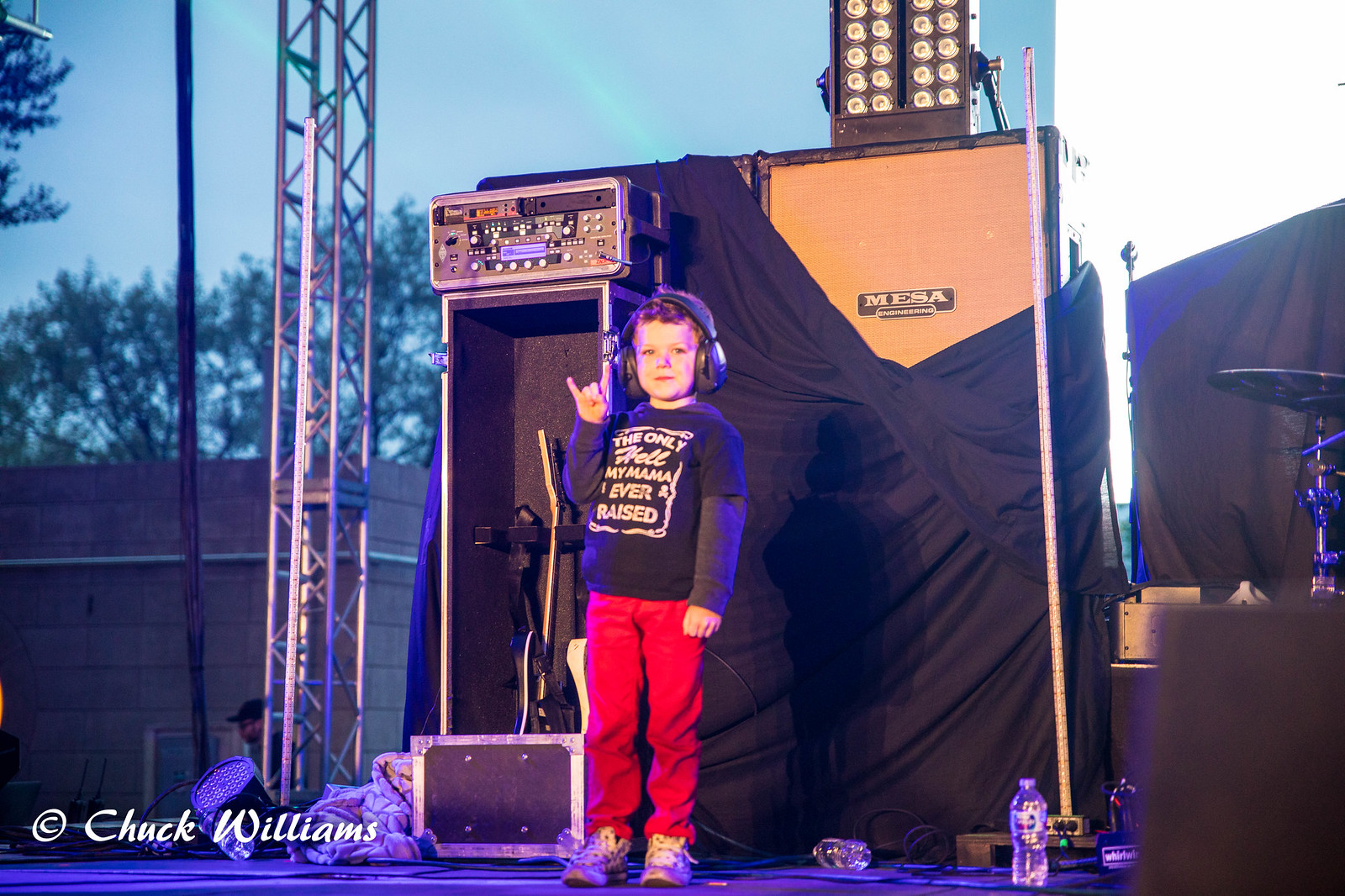In this detailed behind-the-scenes photograph of an outdoor music concert event, a little boy stands confidently in the center of the stage. He has short black hair and wears a long-sleeved black t-shirt layered under a graphic black short-sleeved shirt that reads, "The only hell my mama ever raised." He pairs this with vibrant red pants and tennis shoes. He dons black headphones and makes a 'devil horn' sign with the forefinger and pinky of his right hand held up in front of him, while his left arm rests naturally by his side. Behind him, looming taller than he is, is a large speaker partly covered by a black tarp, with some lights positioned on its right side. To his left in the image, a silver metal tower of scaffolding rises, potentially supporting stage lights. The stage floor near him is strewn with a few empty water bottles, and a cymbal from a drum set is visible to the far right, hinting at a larger band setup. The background features a concrete building wall and additional black tarps covering equipment. An inscription at the bottom left of the image attributes the photo to Chuck Williams. The sky indicates early evening as the sun begins to set, casting a soft glow over the scene.